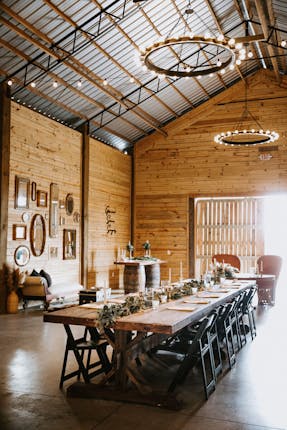The image depicts a color photograph of an elegant banquet setting within a modern, barn-like structure. The building features a corrugated aluminum roof supported by wooden beams and wooden slat walls adorned with framed pictures in various shapes. The main focus is a long table, set for approximately 25-30 people, running centrally through the space, adorned with a garland, candles, and neatly placed napkins and utensils. Black metal or wooden chairs, likely folding, line both sides of the table. On the left side of the image, there is a small table supported by two wooden barrels. The space is illuminated by natural light streaming in through an opening that resembles a sliding barn door, as well as by hanging string lights and two large circular chandeliers with bulbs spread around the perimeter. The overall ambiance suggests a setting perfect for a wedding or celebratory banquet, with attention to rustic and modern details.